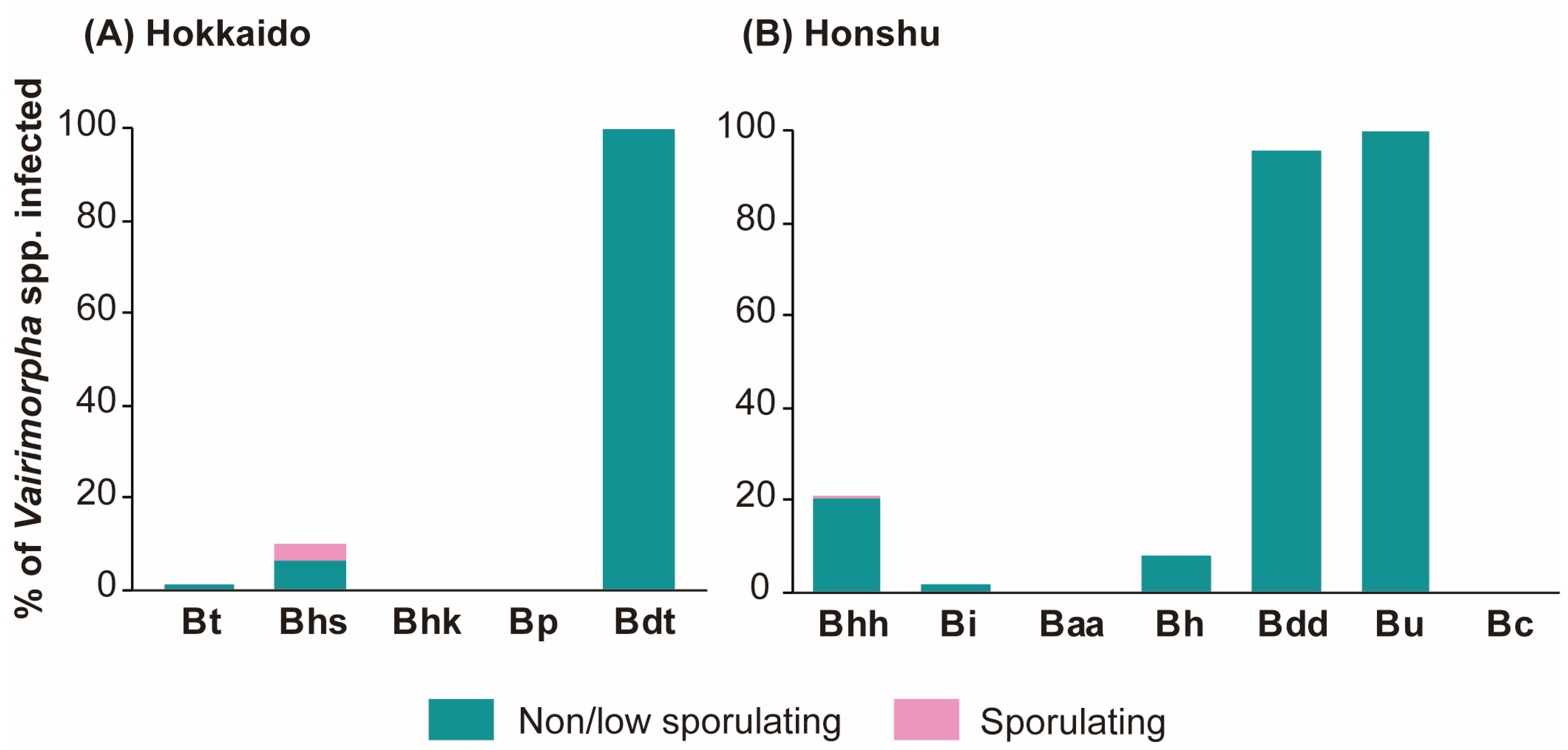The image depicts two bar charts on a white background, each labeled with different regions and measurements. The chart on the left is labeled "A: Hokkaidu" and the chart on the right is labeled "B: Honshu.” 

In the "Hokkaidu" chart, the vertical axis indicates the "Percent of Varimorpha spp. Infected," ranging from 0% to 100%. The horizontal axis is marked with categories: BT, BHS, BHK, BP, and BDT. The chart employs a color-coded key: green bars represent "Non or Low Sporulating," and pink bars signify "Sporulating." The data shows:
- BT: A small green bar.
- BHS: A green bar with a smaller pink section on top.
- BHK: No bars.
- BP: No bars.
- BDT: A tall green bar reaching nearly 100%.

In the "Honshu" chart, the y-axis also measures the "Percent of Varimorpha spp. Infected" with the same scale. The x-axis categories are: BHH, BI, BAA, BH, BDD, BU, and BC. This chart predominantly features green bars, with no significant pink bars. The details are:
- BHH: A green bar up to around 20%, with a minute pink area.
- BI: A very small green bar.
- BAA: No bars.
- BH: A small green bar just above 0%.
- BDD: A green bar reaching slightly above 80%.
- BU: The tallest green bar, slightly longer than BDD.
- BC: No bars.

Overall, the chart highlights the prevalence of non or low sporulating (green) and sporulating (pink) cases across specified categories in two regions, Hokkaidu and Honshu.